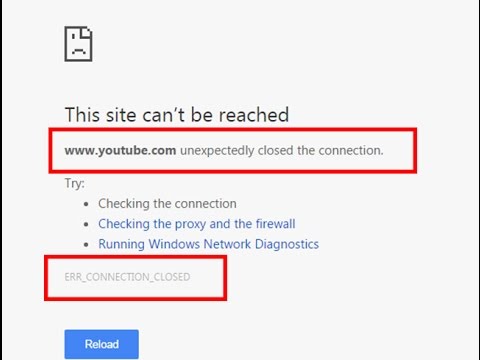The image appears to be a screenshot from a computer displaying a browser error message. In the top left corner, there is a small, pixelated icon of a file with a frowning face. Below the icon, bold black text reads, "This site can't be reached." A red horizontal rectangle highlights the URL "www.youtube.com," accompanied by the message "unexpectedly closed the connection." Beneath this, there are three suggested troubleshooting steps in black text, listed with bullet points. The first step reads, "Checking the connection." The next two steps, in blue text, read, "Checking the proxy and the firewall" and "Running Windows Network Diagnostics."

Further down, another red horizontal rectangle frames a white background with the error code "ERR_CONNECTION_CLOSED" in light gray text. Below this, a small blue horizontal rectangle with a white font contains the word "Reload." The sides of the image are bordered by black lines, creating a semi-frame, while the top and bottom remain unbordered, leading into an off-white gray background that encompasses the entire screen.